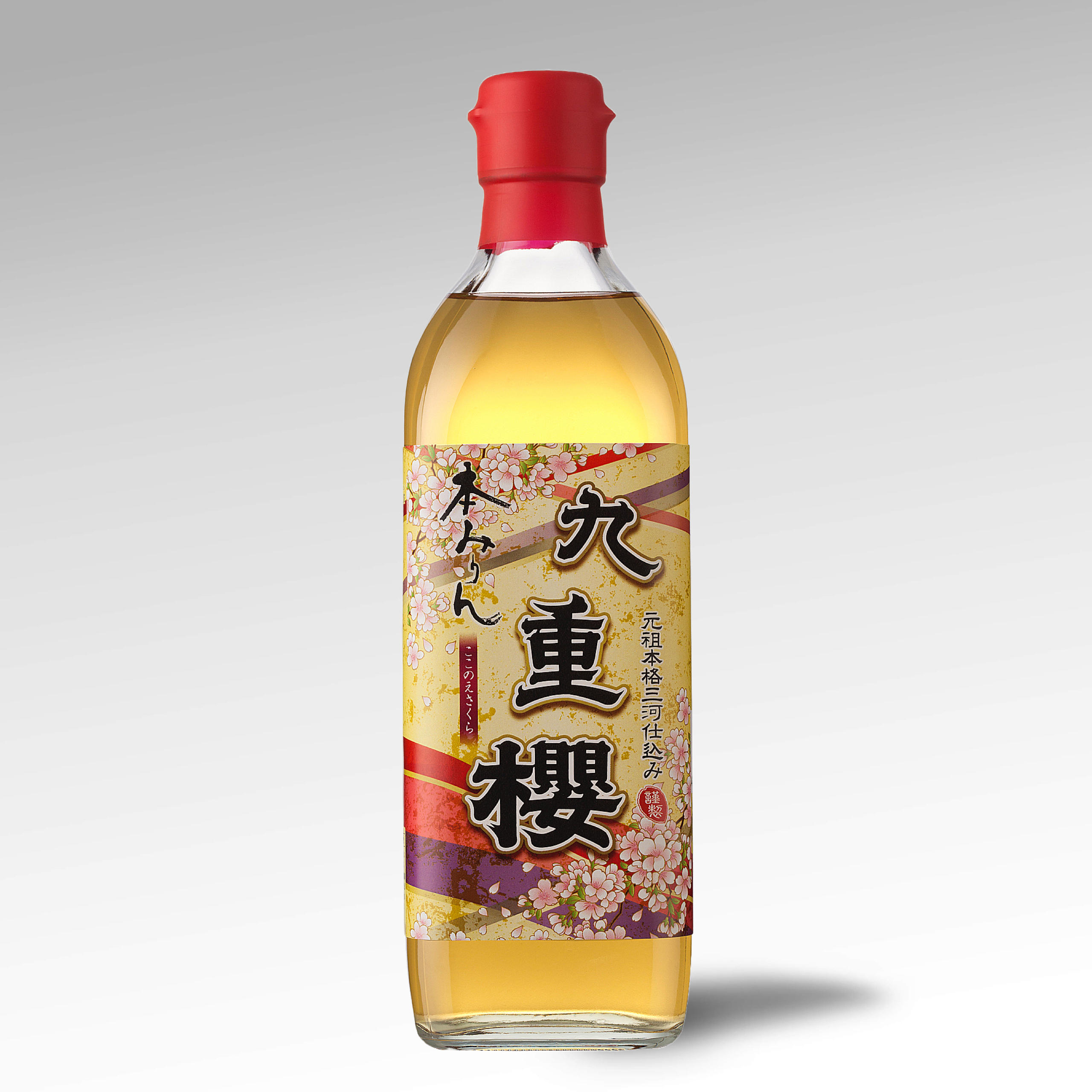The image showcases a clear, one-quart glass bottle with a distinctly autumn-themed label, resting against a gray background. The bottle, sealed with a red wax cap, is filled with a tan liquid reminiscent of beer in color, though it could potentially be an oil or vinegar. The label, adorned with Japanese text, is a medley of warm hues, predominantly various shades of yellow, accented by stripes of purple, burnt orange, and burnt red, enhancing its autumnal feel. Pink cherry blossoms embellish the label in a triangular pattern, emerging from the lower right and upper left corners. The text, primarily vertical, includes both larger and smaller characters, contributing to the sophisticated, yet traditional aesthetic of the product. The overall image, a product photograph, is centered and almost square in shape, emphasizing the bottle’s design and details.